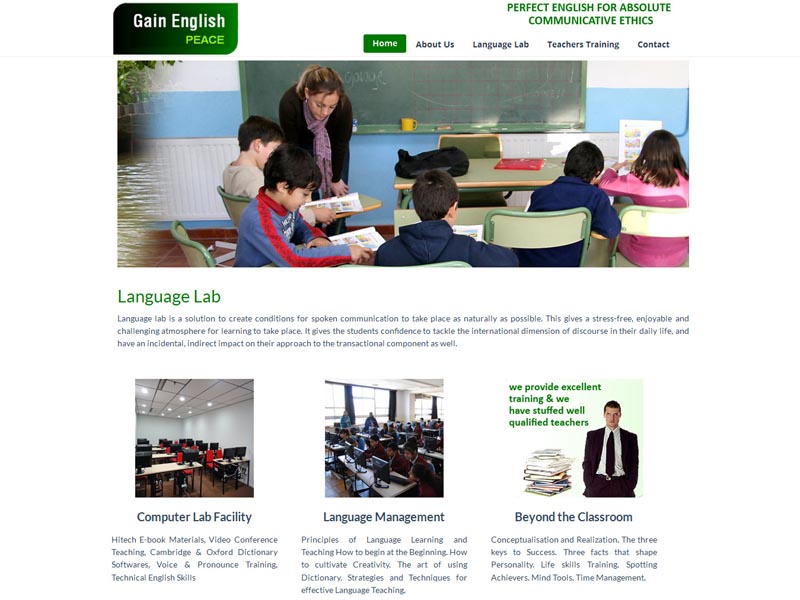**Image Description:**

The image depicts a vertical webpage with a predominantly white background, taken from a computer screen. At the top left corner, the phrase "Gain English" is displayed in a dark-to-light green ombre gradient, with the words in white. Directly beneath it, the word "Peace" is written in a lime green hue. 

In the top right corner, there's a tagline that reads "Perfect English for Absolute Communicative Ethics." Below this tagline, a navigation menu is visible with various clickable options: "Home" (highlighted in green), "About Us," "Language Lab," "Teachers Training," and "Contact" (all in black).

The central part of the image features a photograph of a teacher assisting students. The setting resembles an old-school classroom with small desks and chairs. The teacher, holding a piece of paper, leans over to support one of the five visible students.

Below the image, a green heading titled "Language Lab" introduces a descriptive blurb: "Language Lab is a solution to create conditions for spoken communication to take place as naturally as possible. This gives a stress-free, enjoyable, and challenging atmosphere for learning to take place. It gives the students confidence to tackle the international dimension of discourse in their daily life and have an incidental indirect impact on their approach to the transactional component as well."

Further down, the page mentions additional resources and facilities:
- "Computer Lab Facility"
- "Language Management"
- "Beyond the Classroom"

There's a small icon of a man accompanying the text "we provide excellent training, and we have staffed, well-qualified teachers." Each of these options has associated blurbs, although the specifics are not detailed in this summary.